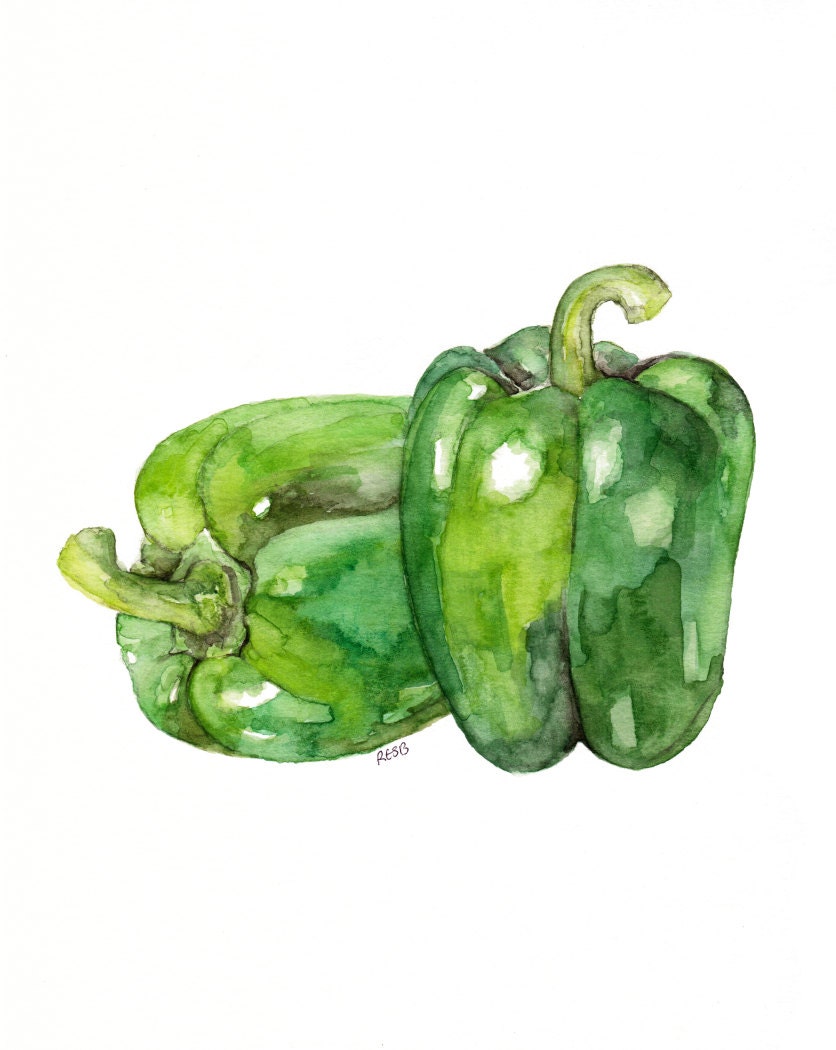The image depicts a realistic watercolor painting of two green bell peppers on a completely white background. One bell pepper is standing upright while the other lies on its side, slightly behind the first. The peppers are a vibrant mix of various shades of green, from light to dark, with white highlights suggesting a reflective surface. The peppers are bordered with darker, almost black lines that enhance their contours and give them a three-dimensional appearance. Near the bottom of the image, there is a signature reading "R.E.S.B," indicating the artist. Overall, the painting is detailed and captures the lifelike quality of the peppers using a nuanced blend of colors and shading.